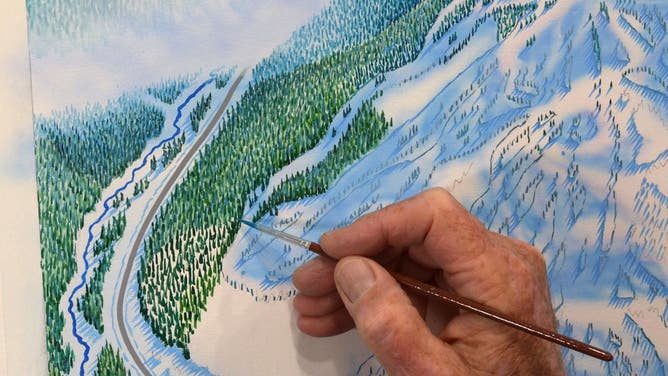In this close-up image, we see an older man's weathered hand holding a very thin paintbrush with a brown handle and a metal tip. He is meticulously painting a detailed landscape on a canvas that lies on a white surface. The canvas captures a serene scene featuring lush green fields and densely packed pine trees. The artist is adding small green trees to a valley that stretches out from a hill. Within the valley, a creek runs through, joining various water paths that wend through the landscape. In the distance, there is a striking snow-capped mountain range, and clouds loom above, adding a sense of depth. The right side of the painting features a gleaming glacier. Notably, a section near the artist’s hand remains unfinished, indicating the ongoing nature of his work.